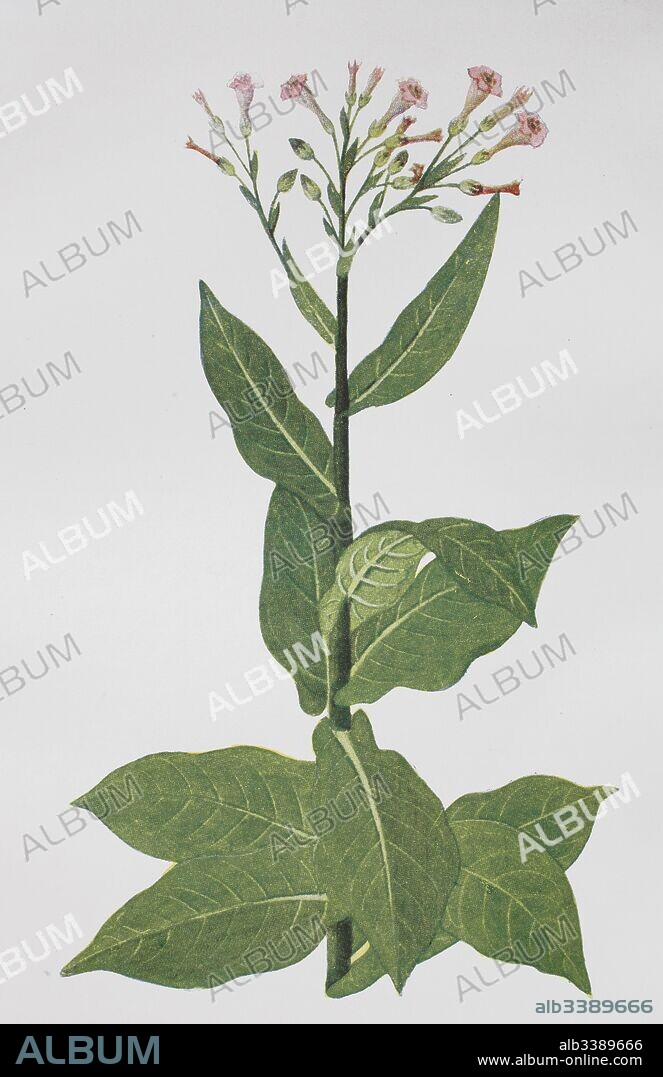The image is a detailed screenshot from the website album-online.com, labeled with the identifier ALB3389666. It features a leafy plant with several prominent green leaves, each bearing distinct white veins. The bottom two-thirds of the plant is dense with these large, tree-like leaves. At the top, the plant showcases budding flowers that resemble tulips, with thin pink petals just beginning to bloom. Some of the buds remain closed, appearing as green teardrop shapes. The image is heavily watermarked with the word "album" in white and gray text across the background, ensuring the picture cannot be stolen. Additionally, the watermark includes the repeated term "album" and the identifier ALB3389666. At the bottom of the image, blue text on a black stripe also says "album," and the website www.album-online.com is displayed in small white lettering on the right. The plant has around twelve leaves and several blossoms that are intricate and vibrant in detail.